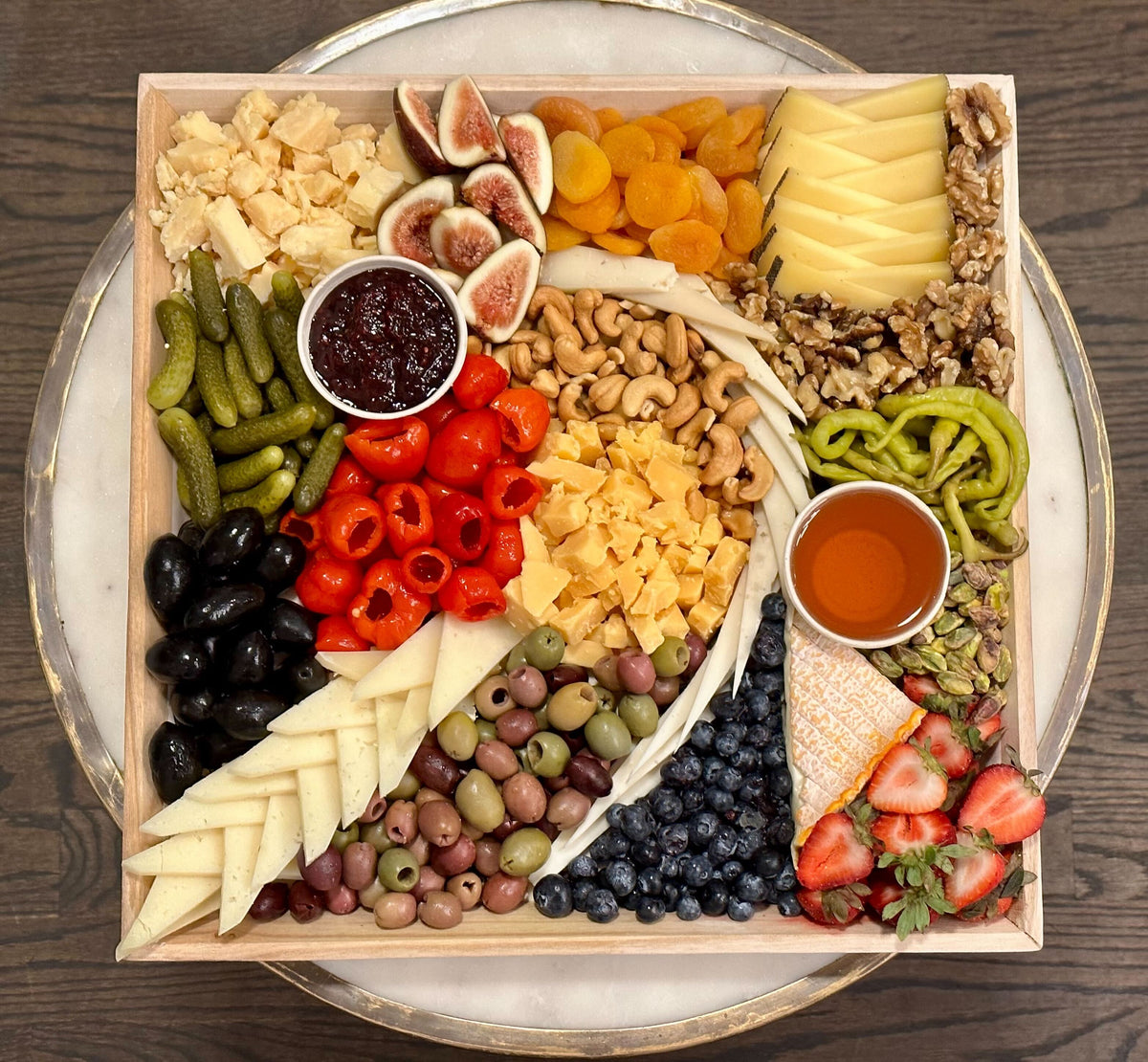The image depicts a charcuterie board, meticulously arranged, displayed on a square, off-white wooden board that sits atop a round white plate trimmed in pewter. Set against a rustic wood panel background, the charcuterie board is an inviting feast of various finger foods. In the upper left corner, small yellowish-beige pieces of cheese stand next to vibrant pieces of fig and slices of dried oranges. Below this, a delightful medley of small gherkin pickles, black olives, and red bell peppers is visible, accompanied by scattered nuts including cashews and pistachios.

More intriguing finds include an assortment of green and purple olives, mixed in with juicy blueberries neatly placed near the center of the board. Two bowls of dipping sauces—one dark brown, possibly a balsamic reduction, and another honey-colored, hinting at a sweet contrast—are strategically placed amongst the foods. The bottom right corner boasts freshly halved strawberries, adding a pop of color next to the array of different nuts and vibrant vegetables such as cherry tomatoes and sliced carrots.

The background setting, a rich black wooden table, accentuates the array of colors and textures, making the appetizer tray—a rich tapestry of diverse, flavorful delights—appear as though it’s ready to be explored and enjoyed.